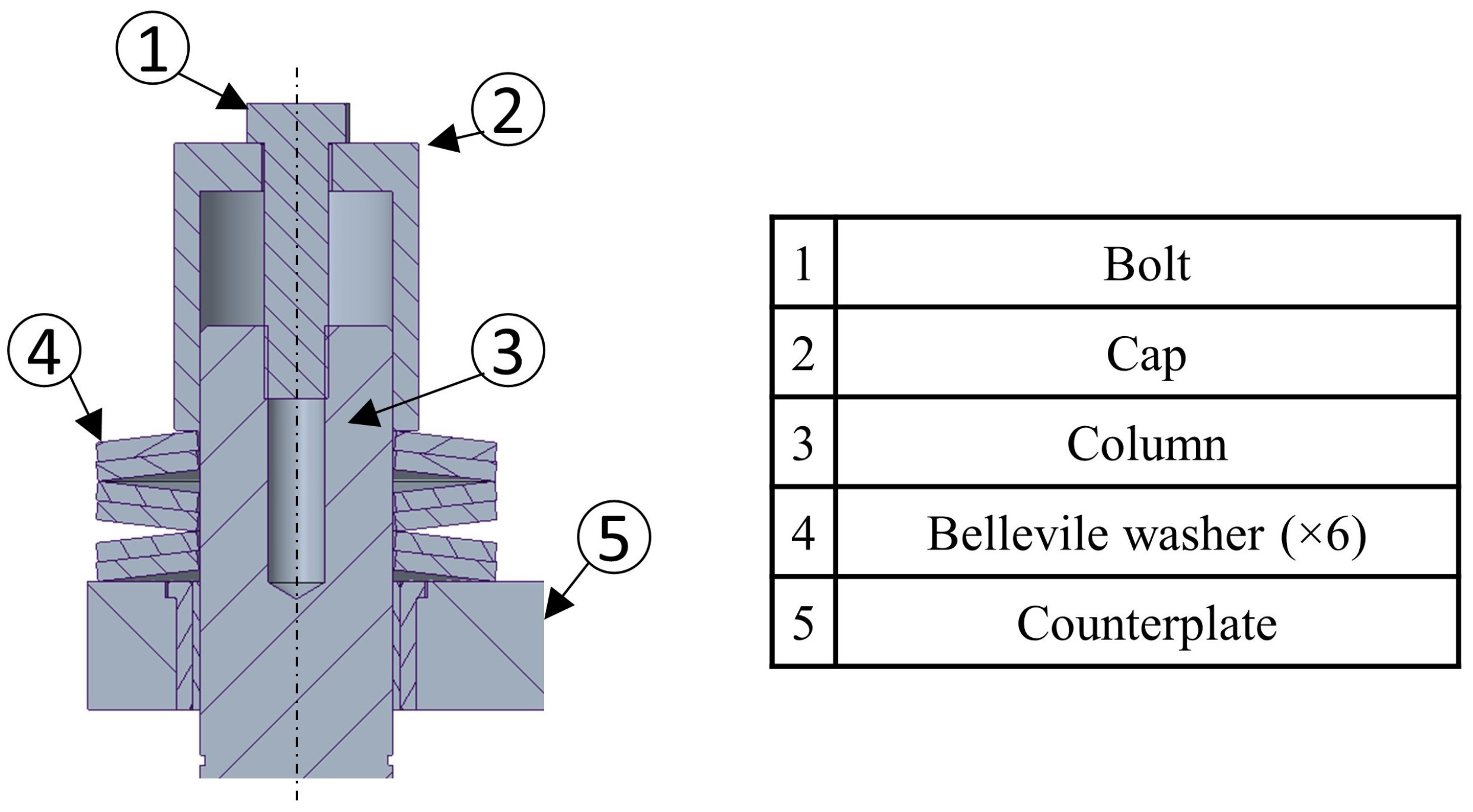The image depicts a detailed assembly diagram for constructing an unidentified item, accompanied by a parts list and identifier table. On the left side of the image, the step-by-step assembly diagram is presented, showing various components labeled with numbers to indicate the order and position of each piece during the assembly process. The diagram itself is rendered in a regular grey color, interspersed with purple lines, the purpose of which is unclear.

On the right side, the image features a comprehensive table that lists and labels each part, specifying both their names and quantities. The components include:

1. Boat
2. Cab
3. Column
4. Belleville washer (quantity: 6)
5. Counterpiece

Each numbered label on the table correlates with corresponding numbers in the assembly diagram, facilitating a clearer understanding of where and how each part should be placed during the construction process. The combination of the visual guide and the part identification table aims to provide a structured and coherent method for assembling the item.